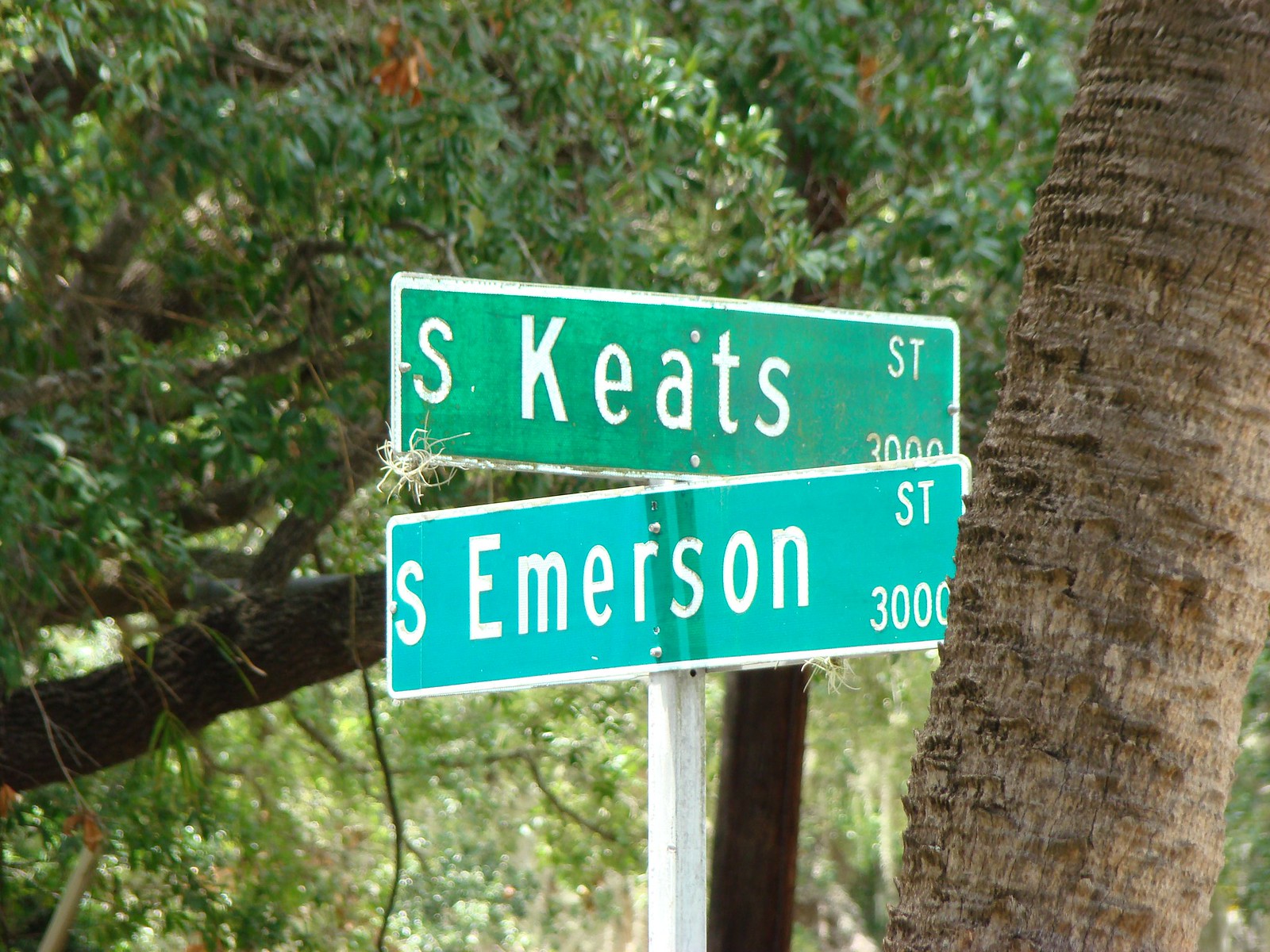A close-up image captures a tall metal pole topped with two intersecting street signs, marking the meeting point of South Keats Street and South Emerson Street. The upper sign, a dark green plate adorned with bold white lettering, announces "South Keats Street," while the lower sign, positioned perpendicularly, is a bluish-green plate also featuring white letters, indicating "South Emerson Street." The pole is situated adjacent to a sizable tree trunk, anchoring the scene with its solid presence. To the left of the signs, another large tree stands tall, its branches and lush green leaves extending outward. In the backdrop, additional tree trunks and verdant foliage create a layered effect, with sunlight filtering through the leaves, casting a warm glow on the rich greenery.